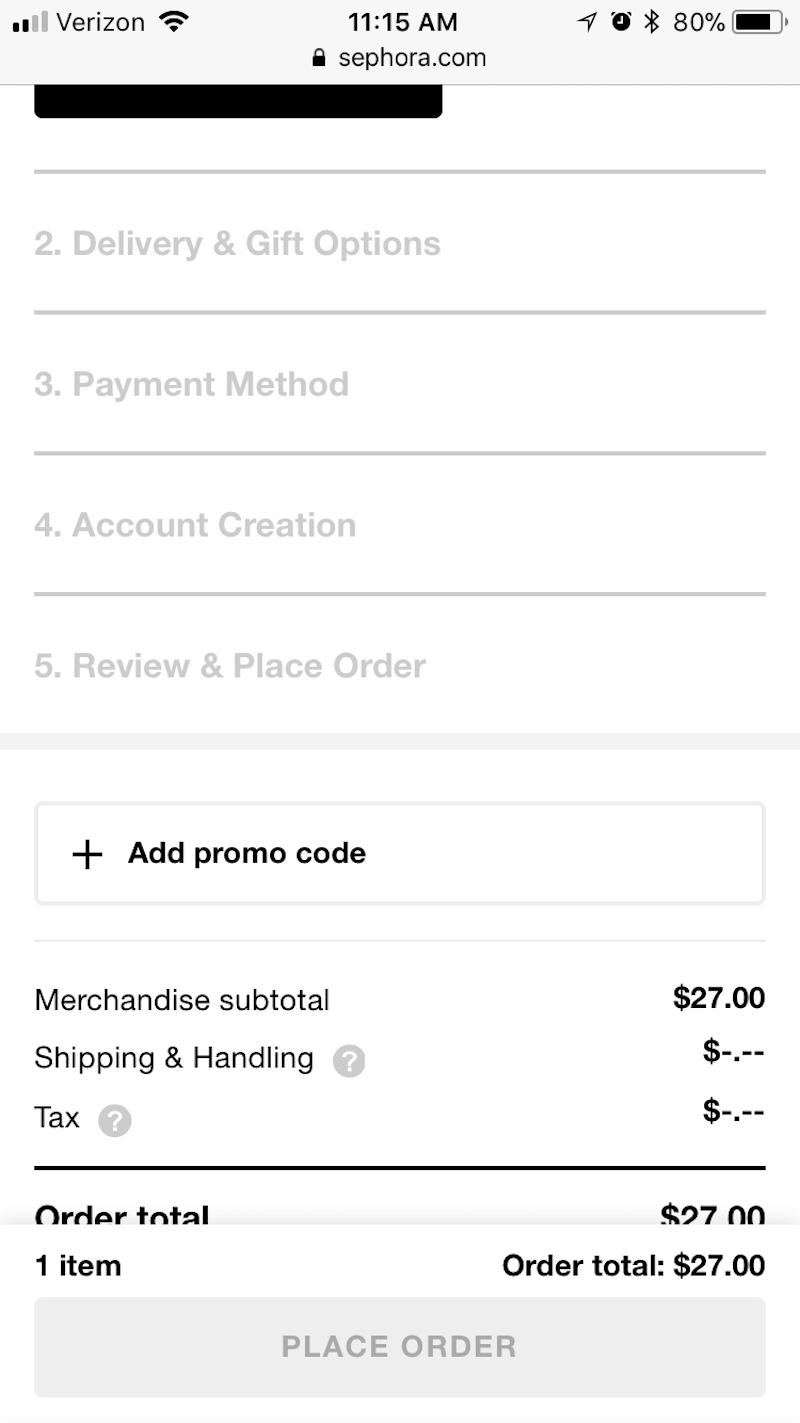The screen displays a digital checkout interface from Sephora.com, featuring a gray border at the top. Within this border, various status icons are visible: Verizon signal strength showing two out of four bars, a Wi-Fi icon, a timestamp of 11:15 a.m., a Bluetooth icon, an 80% battery indicator, and a lock icon. 

Beneath the header, a black box is present, followed by a gray horizontal line demarcating the sections. The step-by-step checkout process is listed:

1. "Delivery and Gift Options," indicated by a header with a line below it.
2. "Payment Method," also marked with a separating line below.
3. "Account Creation" follows, with another dividing line beneath it.
4. "Review and Place Order," separated by yet another line.

Below these steps, a rectangular box invites users to "Add Promo Code," followed by another line. The payment summary section shows the merchandise subtotal as $27, with placeholders for Shipping and Handling and Tax. The order total sums up to $27 for one item, repeated again for clarity as "Order Total: $27." At the bottom of the screen, a gray rectangular button labeled "Place Order" is prominently displayed.